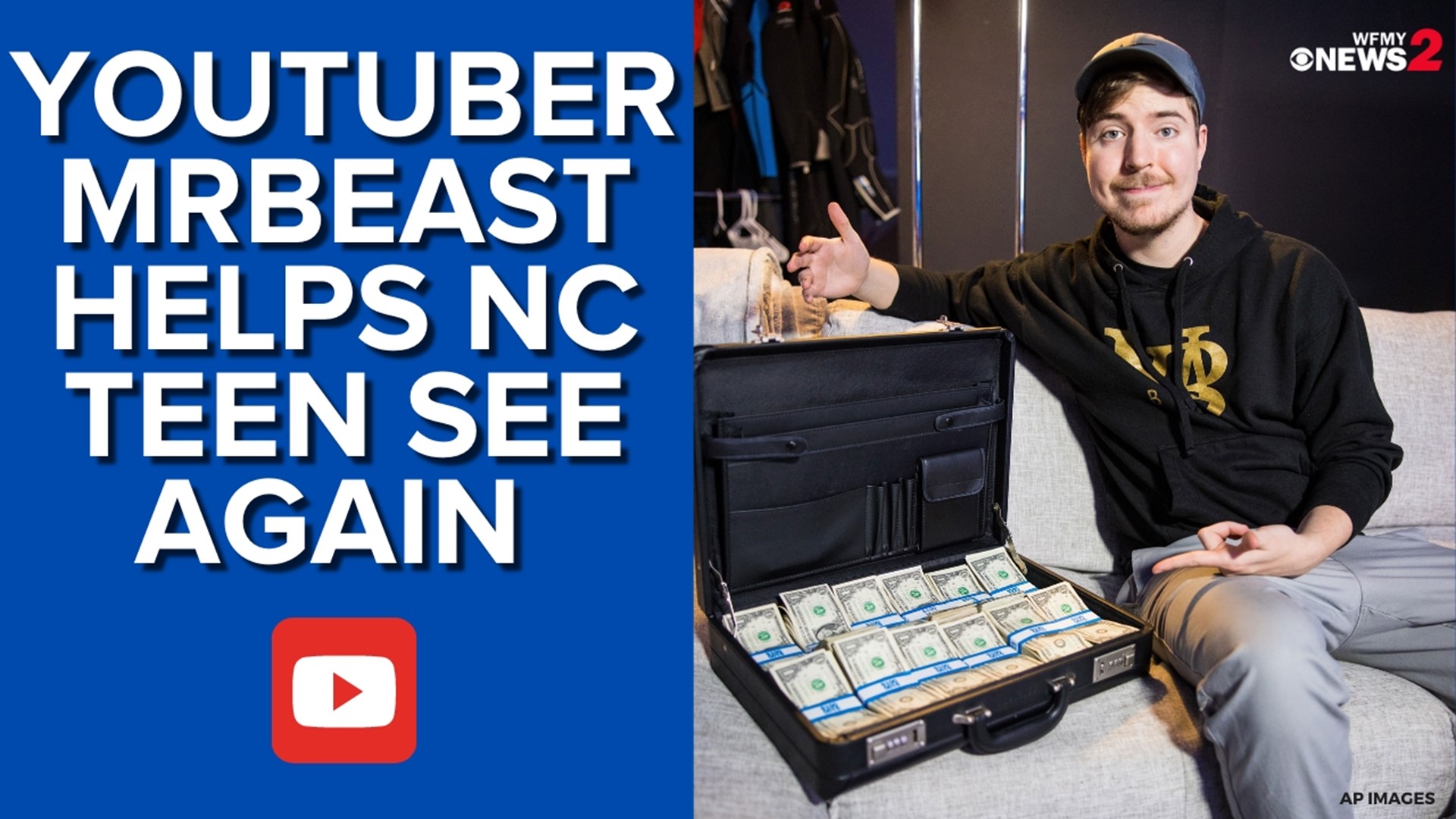The image features a blue background on the left, displaying bold white text that reads "YouTuber MrBeast Helps NC Teen See Again," with a YouTube play button—a red triangle inside a white box—beneath the text. On the right side of the image, a young man with a light beard, mustache, brown hair, and wearing a gray Nike baseball cap, sits on a couch. He is dressed in a black hoodie with gold symbols on the front and gray pants. The man, identified as MrBeast, points towards an open black briefcase filled with tightly bundled stacks of money, each secured with blue wrappers. Above him, the image features the text "WFMY News 2" in white letters and a red numeral against a black background. The background of the entire right side conveys a bright blue hue, adding to the image's vibrant appeal.